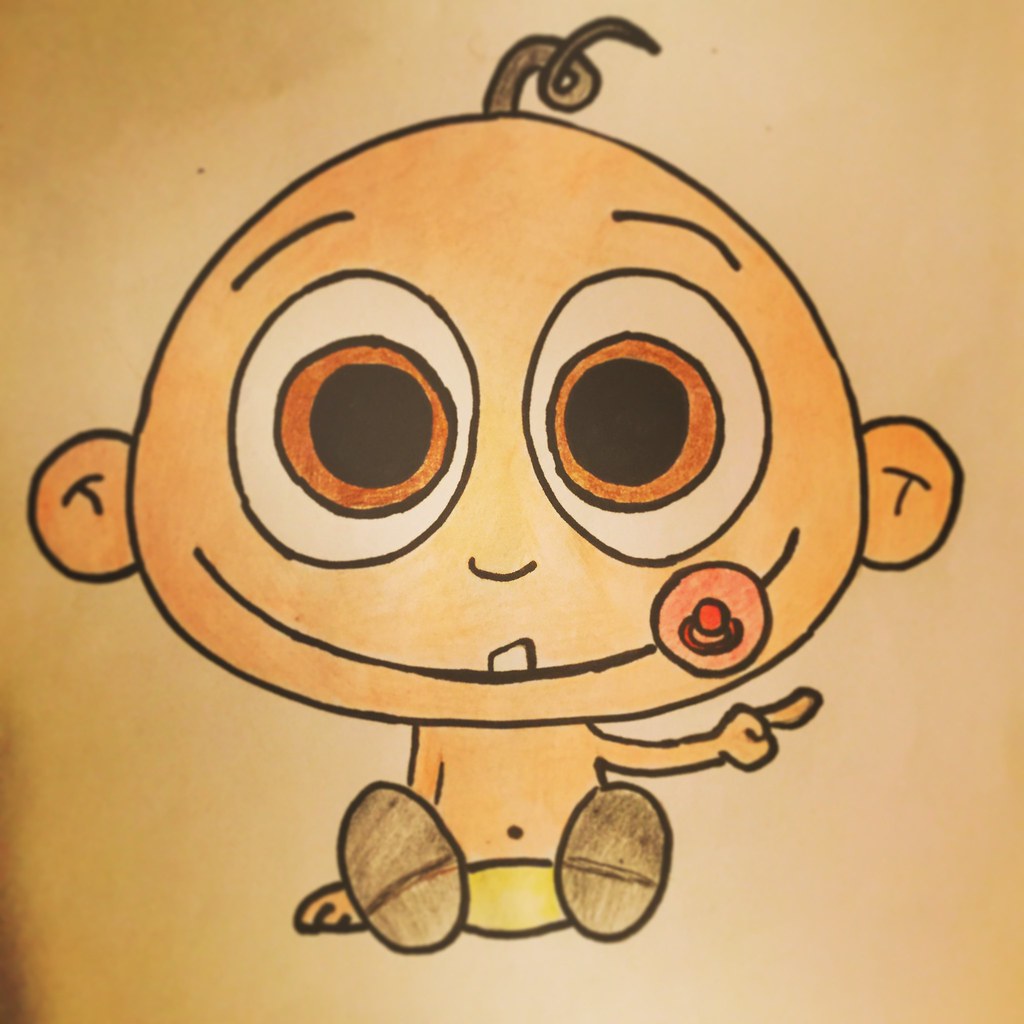This vibrant crayon sketch on cream-colored paper features a whimsical representation of a baby with exaggerated proportions. The baby is depicted with an unusually large, triangular-shaped head that tapers to a rounded point at the top, while the base around the mouth is broad and expressive. The baby's facial features are charmingly playful, with enormous, wide-set eyes resembling brown-irised fried eggs and black pupils, complemented by simplistic lines indicating eyebrows. A single curly hair sprouts adorably from the top of the otherwise bald head.

The mouth, a narrow grin, prominently displays one tooth and is adorned with a red pacifier tucked into the corner. The baby's small torso is clad in a yellow diaper or pants, and its posture suggests a lively demeanor. Seated on the ground, the baby supports itself with its right arm, the hand firmly planted on the surface. The left arm is extended horizontally, with a clenched fist and an extended finger in profile, hinting at a potentially cheeky gesture, though the specific finger is unclear.

The sketch captures the baby in a pair of brown shoes, with a line indicating a heel, visible from the bottom view due to the seated angle. This detailed, imaginative drawing emphasizes the baby's oversized head and eyes, creating a playful and endearing visual narrative.